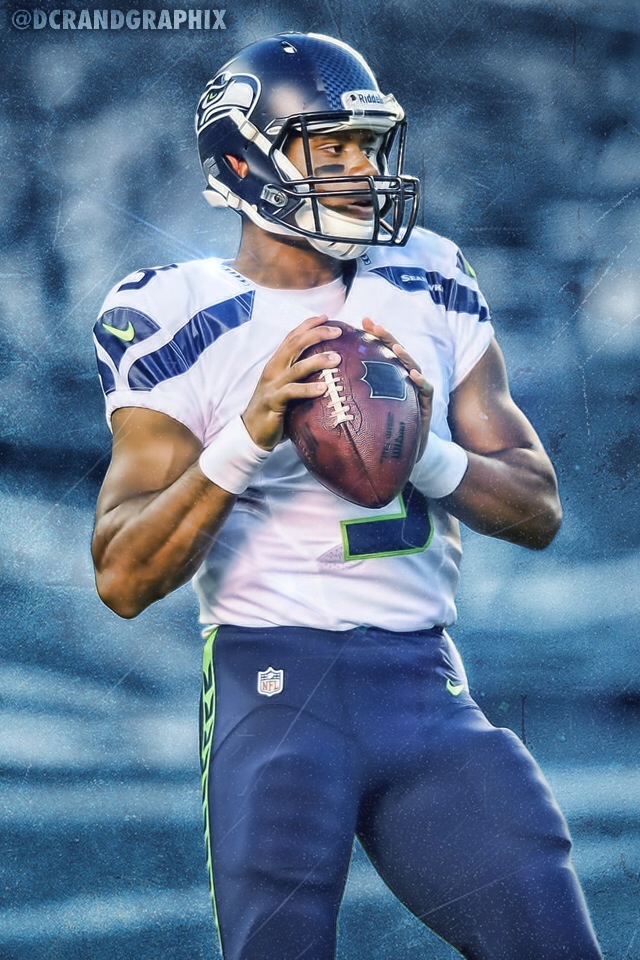The image features a black football player, likely a younger Russell Wilson, who is posing with a football in both hands, preparing to throw a pass. His right hand is wrapped around the laces, and his left hand supports the front of the football. He wears a Seattle Seahawks uniform: a white jersey with blue accents, including stripes below the shoulder pads, and a green-trimmed blue number three on his chest. The jersey also has a distinct green Nike swoosh logo on the right shoulder. He sports dark blue pants with green stripes down the sides and an NFL logo. His helmet is blue with a bird logo on the side, matching his overall team gear. Additionally, he has white wristbands on both wrists. The backdrop is a textured blue, giving the image a weathered appearance, while the upper left corner features the text "@DC Grand Graphics."